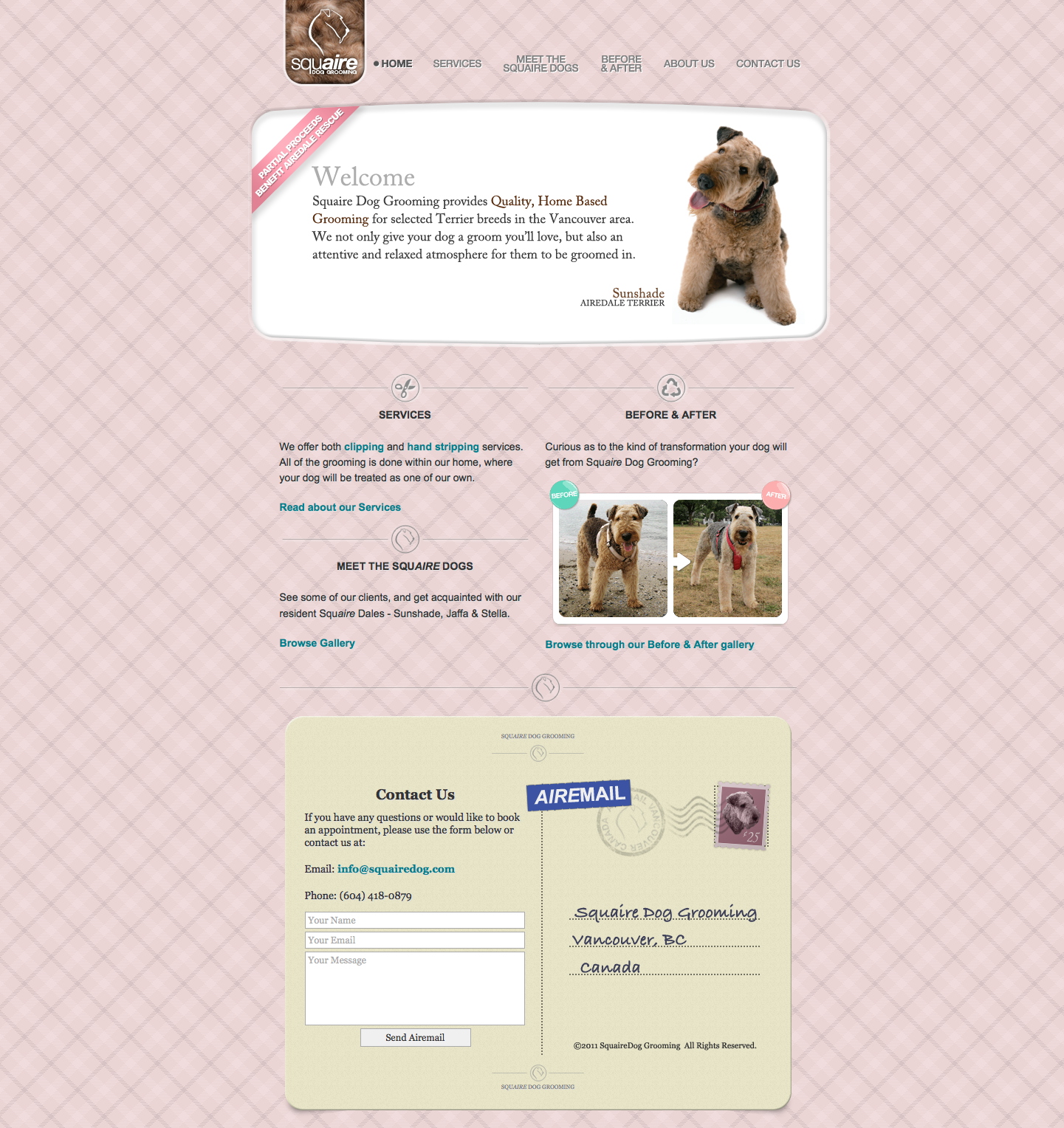This webpage for Square Dog Grooming features a playful background of pink diamonds outlined in gray. In the top left corner, the text "Square" prominently appears, spelled out as "S Q U A I R E." Adjacent to this, the navigation menu includes links to "Home," "Services," "Meet the Soulmate Dogs," "Before and After," "About Us," and "Contact Us," all rendered in a sleek gray font.

Beneath the menu, a horizontal white rectangle greets visitors with the word "Welcome" inscribed in gray. This section elaborates: "Square Dog Grooming provides quality home-based grooming for long-haired terrier breeds in the Vancouver area. We not only give your dog a groom you'll love, but also create an attractive and relaxed atmosphere for them to be groomed in." A picture of a fluffy terrier accompanies this welcoming note, showcasing the grooming services offered.

The "Services" section immediately follows, highlighting their offerings: baths, clipping, and stripping services, all performed within the comfort of their home environment for a more personalized experience. Below this text, two images illustrate a "Before and After" transformation, showing a terrier with poofy hair beside a neatly groomed counterpart.

The page concludes with what resembles a postcard, featuring the "Contact Us" section for any inquiries or appointments.